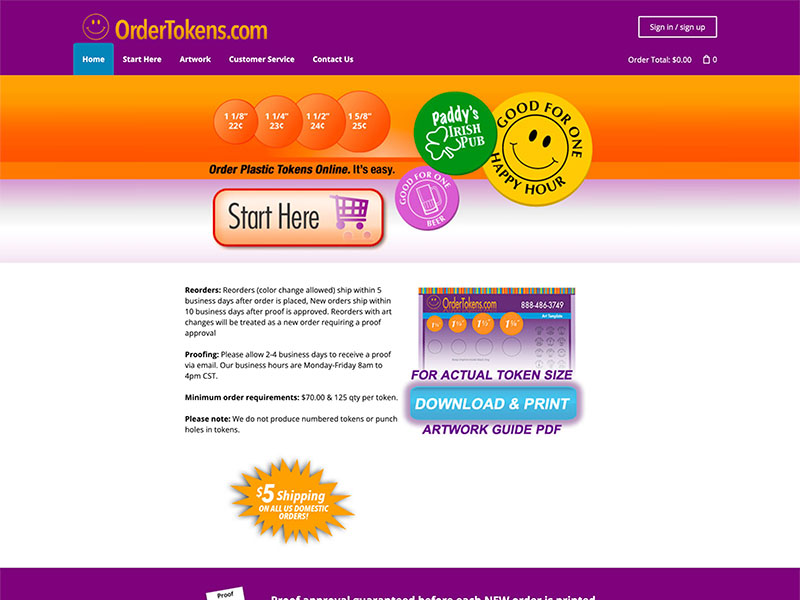This screenshot captures the homepage of the website OrderTokens.com, showcasing a user-friendly interface compatible with desktop, laptop, and tablet devices. The main background is predominantly white, while the design features vibrant purple banners at both the top and bottom of the page. Just beneath the top purple banner, an orange banner adds a pop of additional color.

Several icons resembling location pins subtly introduce a playful aesthetic. Notably, a green pin with a clover bears the text "Patty's Irish Pub," while a yellow pin, adorned with a smiley face, reads "Good for one happy hour."

Clear, informative descriptions guide users in understanding the website’s purpose – to facilitate easy online ordering of plastic tokens. The site presents various token dimensions and associated costs, with a prominent button labeled "Start Here" next to a shopping cart icon, inviting users to commence their purchase.

Towards the bottom, additional instructions and details elucidate the process further, ensuring a smooth user experience. A standout feature is the bonus banner announcing "$5 shipping on all US domestic orders," providing an attractive incentive for potential buyers.